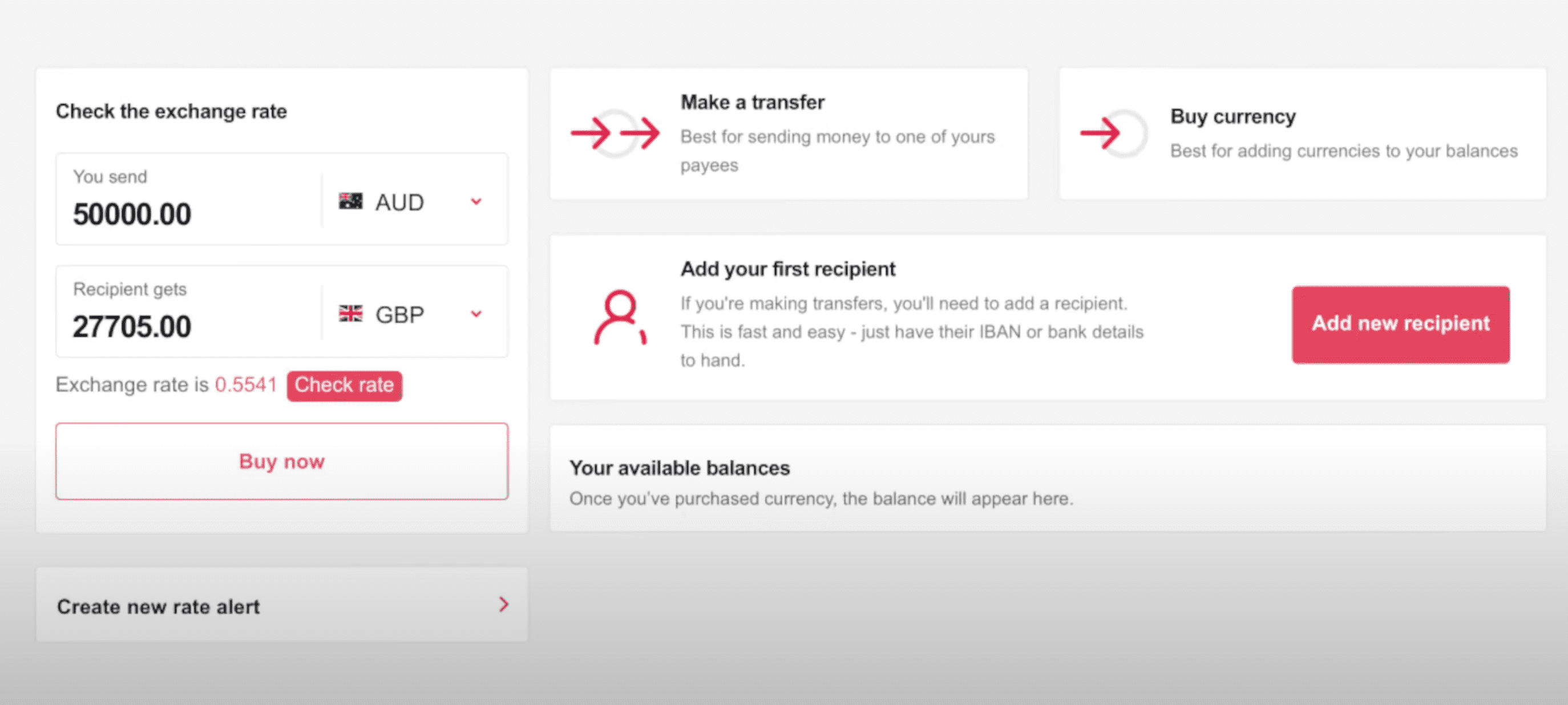This screenshot depicts the interface of a financial application or web page. The layout is horizontally oriented with three primary columns.

1. **Exchange Rate Information:**
   - At the top, the section is titled "Check the Exchange Rate."
   - The first row states, "You send 50,000."
   - The next row specifies the currency as "50,000 AUD" (Australian Dollars).
   - The subsequent row indicates, "Recipient gets 27,705 GBP" (British Pounds), with an exchange rate provided as "0.5541."
   - Additionally, there is an option to "Check Rate" or "Buy Now."

2. **Transfer Section:**
   - The second column is labeled "Make a Transfer."
   - It includes a button that users can interact with to perform a transfer.

3. **Currency Purchase:**
   - The third column begins with the header "Buy Currency."

Beneath these headings are two rows that span across the second and third columns:

- The first combined row prompts the user to "Add your first recipient."
- The second combined row shows "Your available balances."

At the very bottom, there is a clickable link noted as "Create a New Rate Alert."

This detailed breakdown helps in understanding the different functionalities offered by the application at a glance.